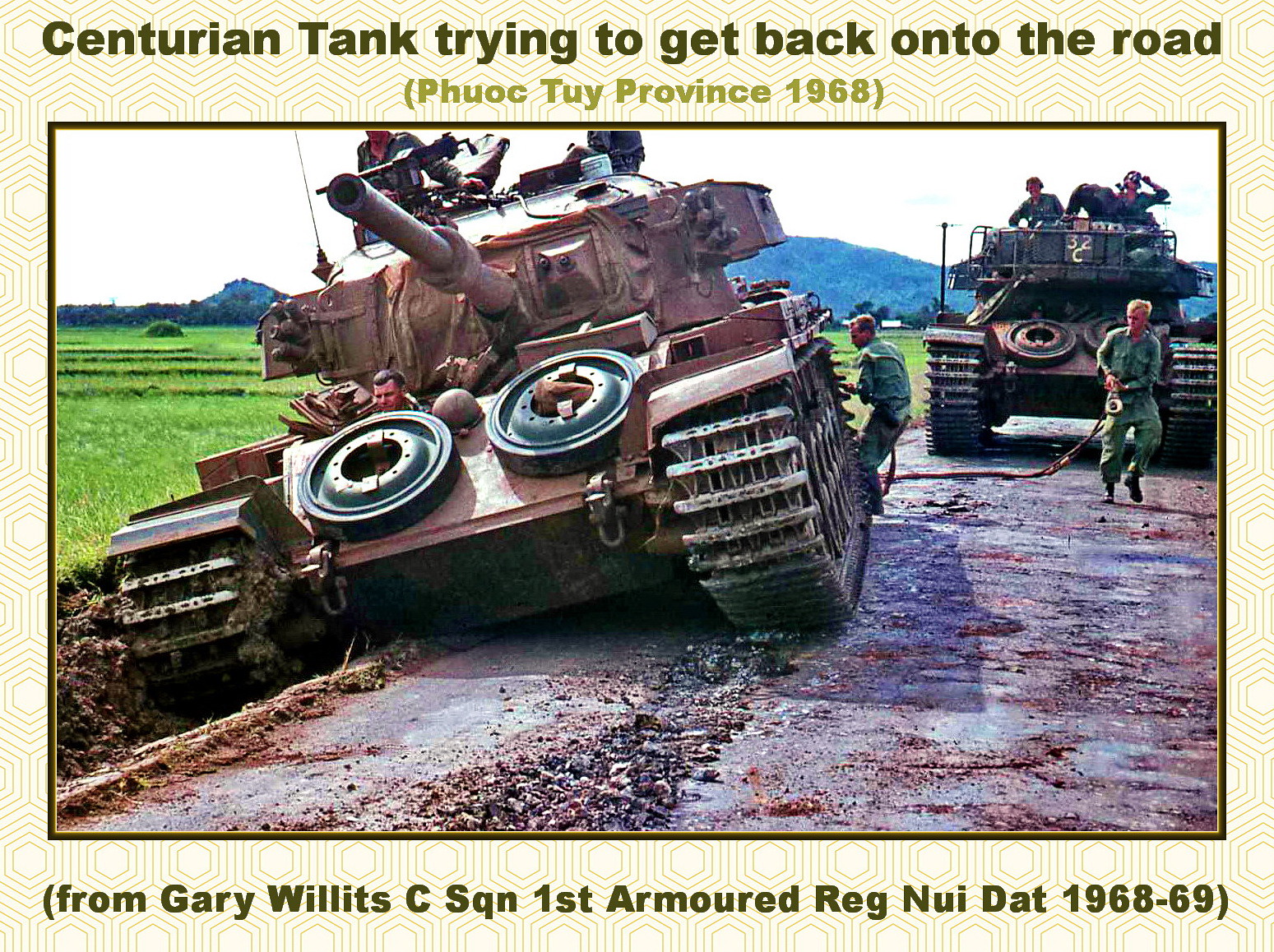In this detailed and dynamic image taken during the Vietnam War, a Centurion tank is depicted stuck halfway in a ditch at the side of a road in Phuoc Tuy Province, 1968. The tank, colored in shades of brown, is surrounded by soldiers; one is seen sitting near the gunner on top, while another climbs the large wheel part. Additional soldiers are visible to the right, seemingly aiding in efforts to extricate the tank. In the background, a large green field and a picturesque mountain range stretch under a mostly white, illuminated sky. Another tank, successfully on the road, is discernible behind, with two individuals seated atop it. The composition of the image is enclosed within a repeating hexagonal yellow border, annotated with captions: "Centurion tank trying to get back onto the road" at the top, and "From Gary Willetts, C-Squadron, 1st Armored Regiment, Nui Dat, 1968-69" at the bottom.